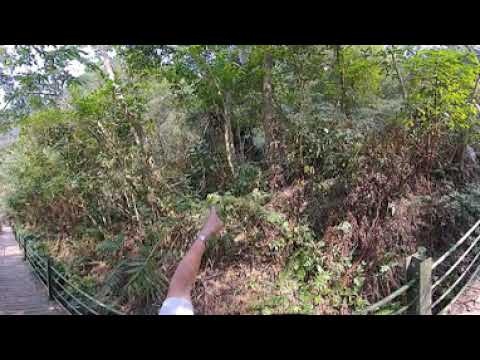This outdoor photograph captures a lush, green forest scene bordered by a wooden and wire fence. Amidst the dense greenery, which includes a variety of trees, shrubs, and bushes, some vegetation shows signs of dryness with a mix of green and dead leaves. A paved walkway or hiking trail encircles the forested area, highlighted by the sunlight dappling through the foliage. Prominently featured in the image is a person's left arm, clad in a white t-shirt and adorned with a silver watch, stretching out and pointing towards the trees and bushes. This arm, belonging to a likely male subject, adds a human element against the backdrop of the verdant yet slightly wilted landscape. The serene scene is softly lit with glimpses of the sky peeking through the canopy overhead.